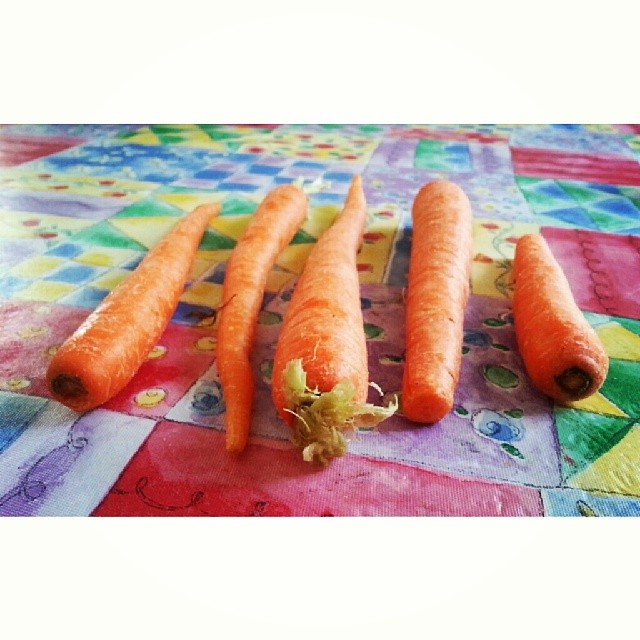This detailed horizontal rectangular photograph captures five vibrant orange carrots meticulously aligned across the center against a distinctive, colorful backdrop reminiscent of a quilt. The multicolored fabric boasts various intricate designs in squares, including checkered, diamond, and floral patterns in shades of purple, red, yellow, green, and blue.

The carrots are positioned horizontally, evenly spaced with their orientations alternating to create visual balance. Starting from the left, the first carrot lies with its thicker end, which features a small black circle, facing the viewer. The second carrot has its pointed, thinner end directed towards the viewer. The third carrot is notable for its cream-colored, frayed top with some greenery still attached, emphasizing it has not been fully trimmed; its thicker end is closer to the viewer. The fourth carrot, which seems almost symmetrical, has its thinner end facing the viewer. Meanwhile, the fifth and final carrot mirrors the first, presenting its thicker end with a distinct black ring where the top was removed.

Natural daylight enhances the texture and organic appeal of the carrots, while highlighting the diversity and vibrancy of the quilt-like backdrop, creating a harmonious and visually pleasing composition.